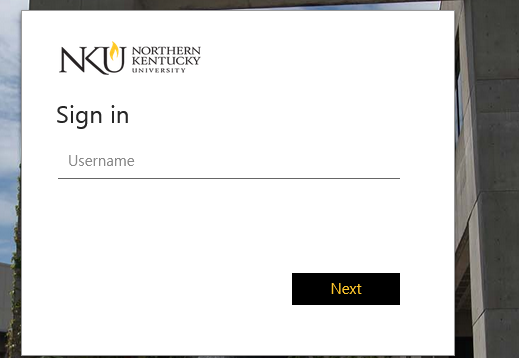Screenshot of the Northern Kentucky University Sign-In Page: 

This image captures the sign-in page for Northern Kentucky University's online portal. At the top left corner is the stylized NKU logo, characterized by a flame motif over the 'K' and accompanied by the full name, "Northern Kentucky University," beneath the letters. Below the logo, a bold heading reads "Sign In," guiding users towards the sign-in prompt.

This prompt includes a username text input field labeled "Username," with an underline indicating where users should enter their credentials. Positioned below the input field is a distinctive "Next" button, featuring a sleek design—predominantly black with a yellow interior—used for proceeding to the next step of the sign-in process after entering the username.

The background of the page is partially visible, showing what seems to be a concrete building or structure, likely part of the university's campus, contributing to the clean and straightforward design of the portal. This page is intended for use by students and staff accessing Northern Kentucky University's web services.